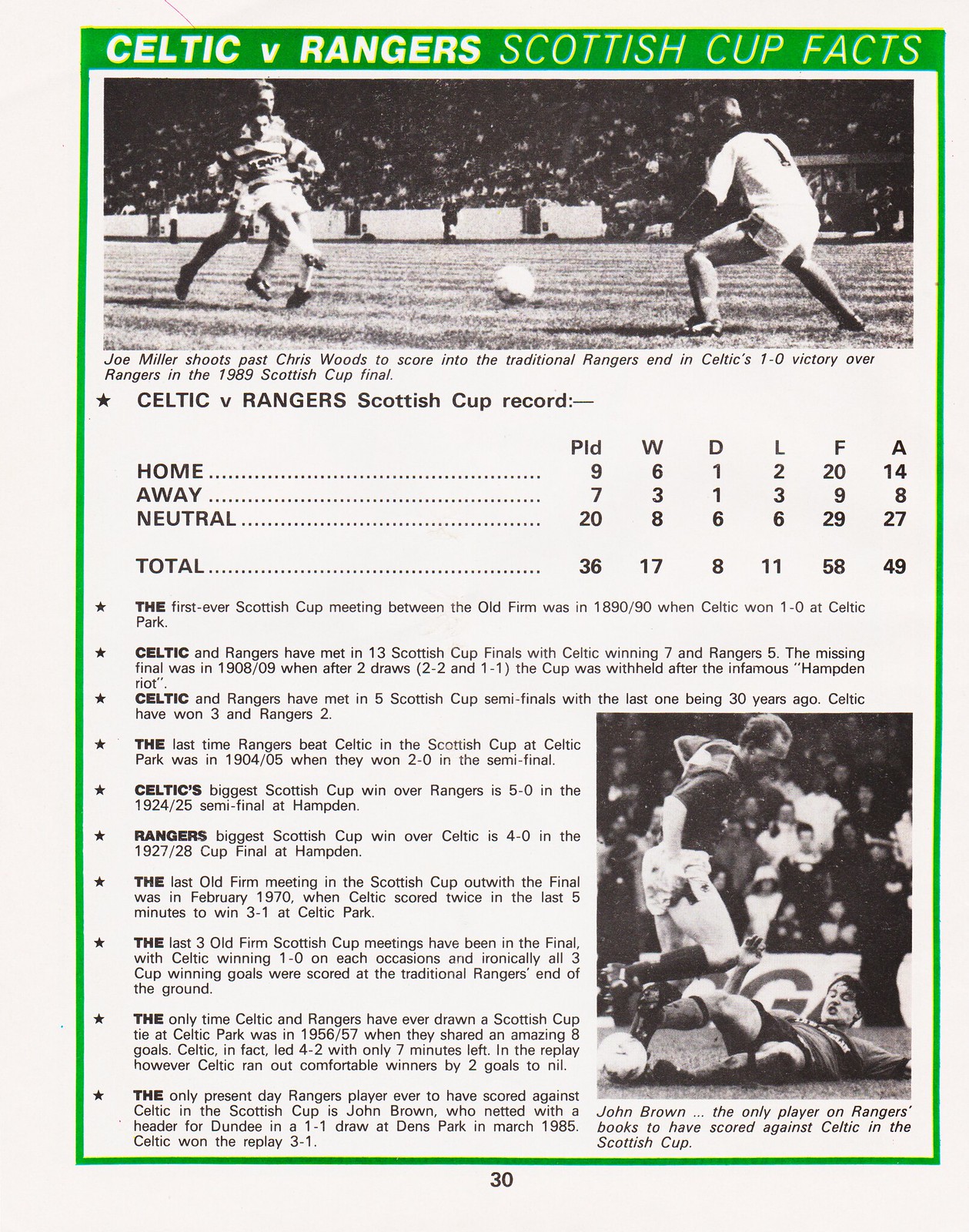This detailed image showcases a fact sheet for a soccer game, bordered with green on an off-white background. At the top, the green border contains white text reading "Celtic versus Ranger Scottish Cup Facts." Below, there's a prominent black-and-white photograph depicting Joe Miller shooting the ball past Chris Woods, contributing to Celtic's 1-0 victory over Rangers in the 1989 Scottish Cup Final. The caption beneath the photo highlights this moment. Further down, the fact sheet details the "Celtic versus Ranger Scottish Cup Record" with columns for home, away, neutral venues, and overall totals. The sheet includes several bullet points elaborating on various statistics. In the lower right corner, there's another image featuring John Brown, noted as the only player on the Rangers' roster to have scored against Celtic in the Scottish Cup. At the very bottom center of the page, the number "30" is written in black text, indicating the page number.